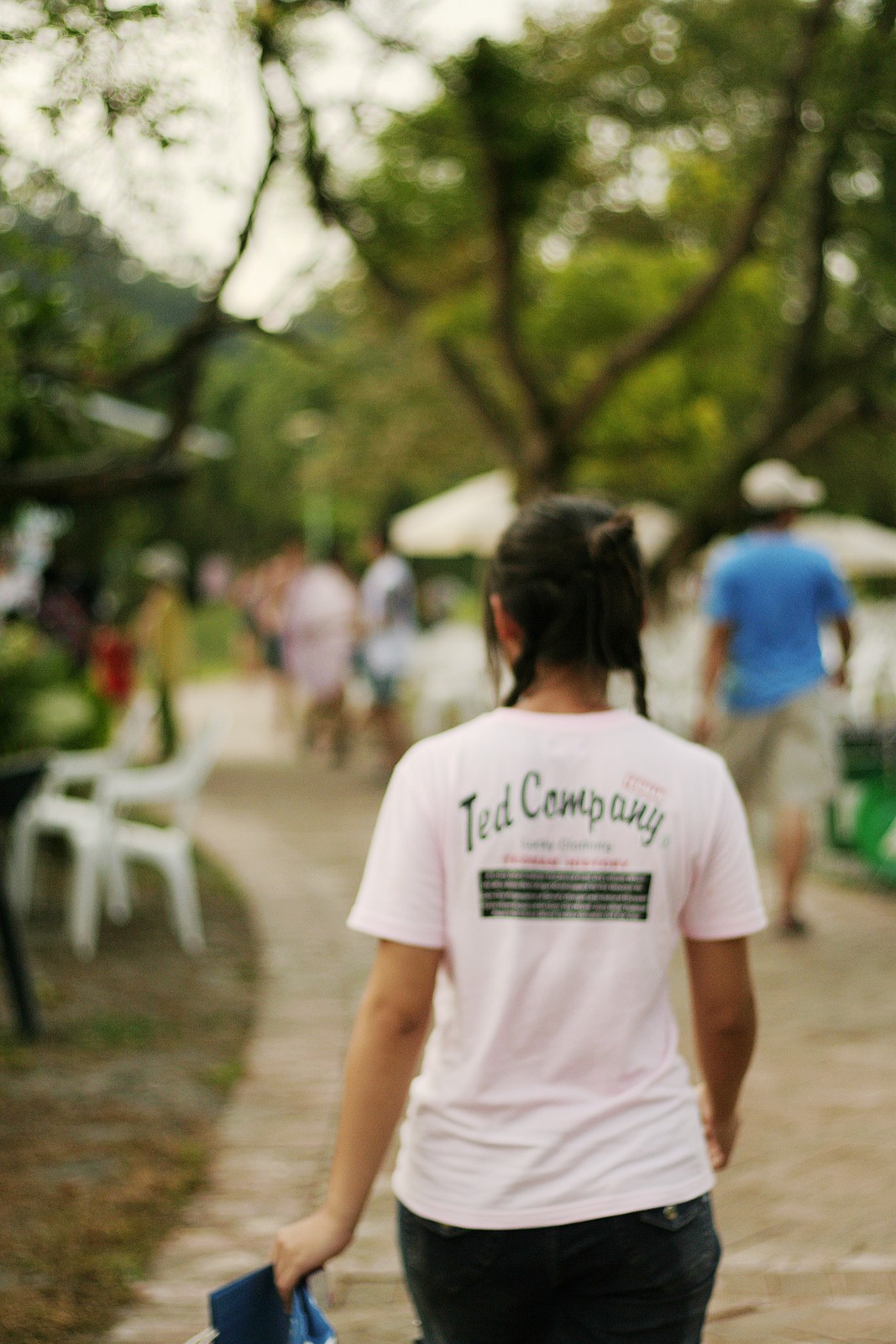This image captures a woman walking away from the camera along a stone or brick walkway in a park-like setting. She stands out in the photo, wearing a very pale pink t-shirt with the words "TED Company" on the back, accompanied by unreadable smaller text. Her dark jeans complement the t-shirt. The woman has medium tan skin, and her hair is styled with the top half in a bun and the bottom half in braided pigtails that hang around the back of her neck. She holds something blue in her left hand. 

In front of her, a man dressed in a blue shirt, khaki cargo shorts, and a white cap is also walking along the path. The background is filled with vibrant green trees and appears slightly overcast, as the sky is mostly white. There are white lawn chairs and umbrellas visible, suggesting seating areas on either side of the walkway, adding to the park atmosphere. The rest of the people and elements are blurred, emphasizing the woman as the focal point.